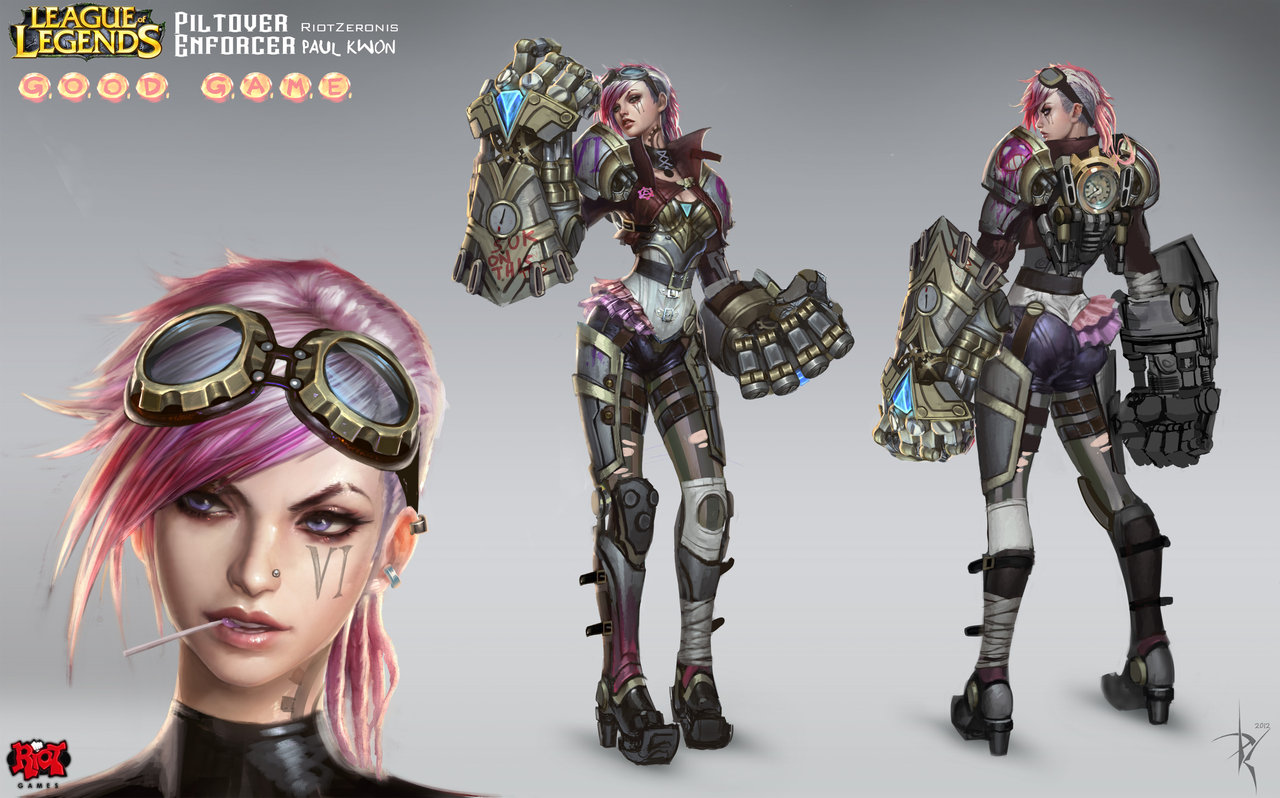This detailed advertisement for the "Piltover Enforcer" skin in the video game League of Legends prominently features the character in three different poses. The upper left of the image is adorned with the League of Legends logo in gold letters, accompanied by the title "Piltover Enforcer" in white. Below, the artist's credit "Riot Zeronis, Paul Kwon" appears in smaller white text, and a faded orange-reddish caption reads "Good Game," surrounded by white circles. 

On the left, the character's face is prominently displayed, showcasing her purple hair and brass, old steampunk-style goggles. Her blue eyes are striking, and a tattoo of Roman numeral VI is etched beneath her left eye. She has meticulously trimmed eyebrows and heavy eyeshadow, with a piercing in her left nostril and a toothpick protruding from her pink lips. A gear tattoo is visible on her neck, and she's clad in a sleek black bodysuit.

The central figure presents her in full battle attire. She dons a corset-like armor, complemented by massive bionic gauntlets that are three to four times the size of her arms and adorned with a large blue triangular crystal on the back of her hand. She sports armor down her legs that protects her kneecaps and shins and heeled black boots with purple accents. 

On the right, the character is depicted from the back, revealing additional details like the purple number 7 on her left shoulder pad. The entire set is rendered in an off-white void with shadowing, ensuring the intricate design elements and cyberpunk-fantasy styling of her thin armor and colossal gauntlets stand out.

A watermark "PK" in the lower right corner credits the artist, Paul Kwon, for this dynamic and intricately detailed skin's design.